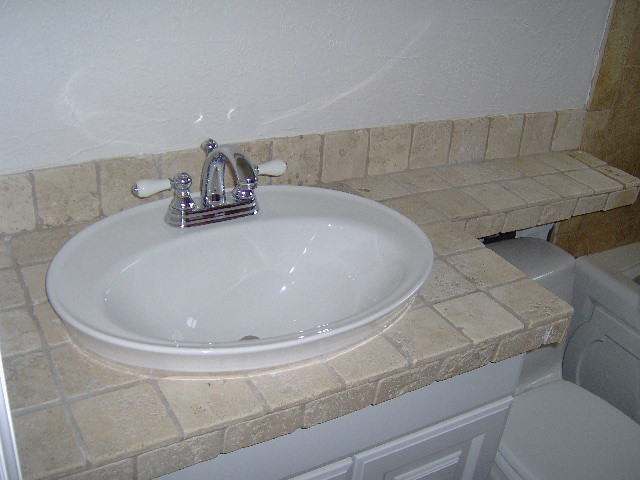This image depicts a bathroom sink and the surrounding counter area. The sink, made of white porcelain, features silver fixtures with handles accented in white at their tips. The sink is slightly raised above the countertop. The countertop, along with the wall area connecting to the sink, is covered in uniform square tiles that extend upward along the wall and horizontally across the entire counter. 

To the right of the sink, a glimpse of a toilet is visible in the corner, along with part of a porcelain bathtub situated next to the toilet, indicating a compact bathroom layout. Below the counter, there is a white cabinet with two drawers; the right drawer is more visible, while the left is partially obscured. The backdrop of the image features a white-tiled wall, contributing to the room's clean and cohesive aesthetic.